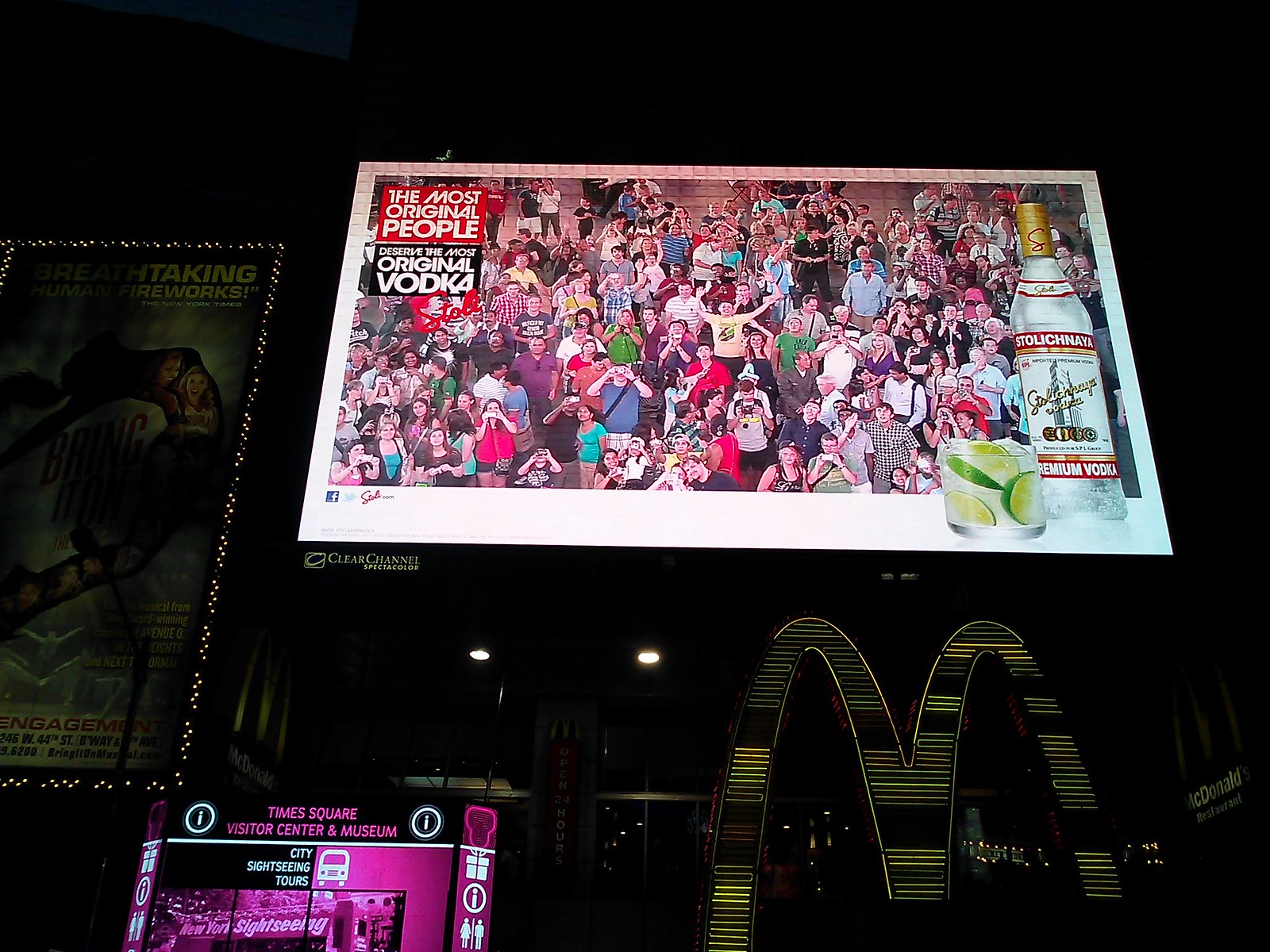This nighttime, landscape-oriented color photograph captures a second-story billboard advertisement prominently featuring a bottle of Stolichnaya Premium Vodka on the right, accentuated by a gold bottle top. Adjacent to the bottle is a glass filled with vodka, ice cubes, and lime wedges. The billboard, bordered by white, showcases a dark background filled with a crowd of people standing and looking forward, as though they are in an audience in a stadium. In the middle of the billboard, "Stola Chania Vodka" is written in gold, accompanied by a white label depicting a white building behind the text. At the top left, a red and black graphic with white text proclaims, "The Most Original People," followed by "Original Vodka." Below the billboard, the illuminated golden arches of McDonald's are visible, and at the bottom left, pink lettering reveals a marquee that reads "Times Square Visitor Center and Museum" in photographic representational realism style.